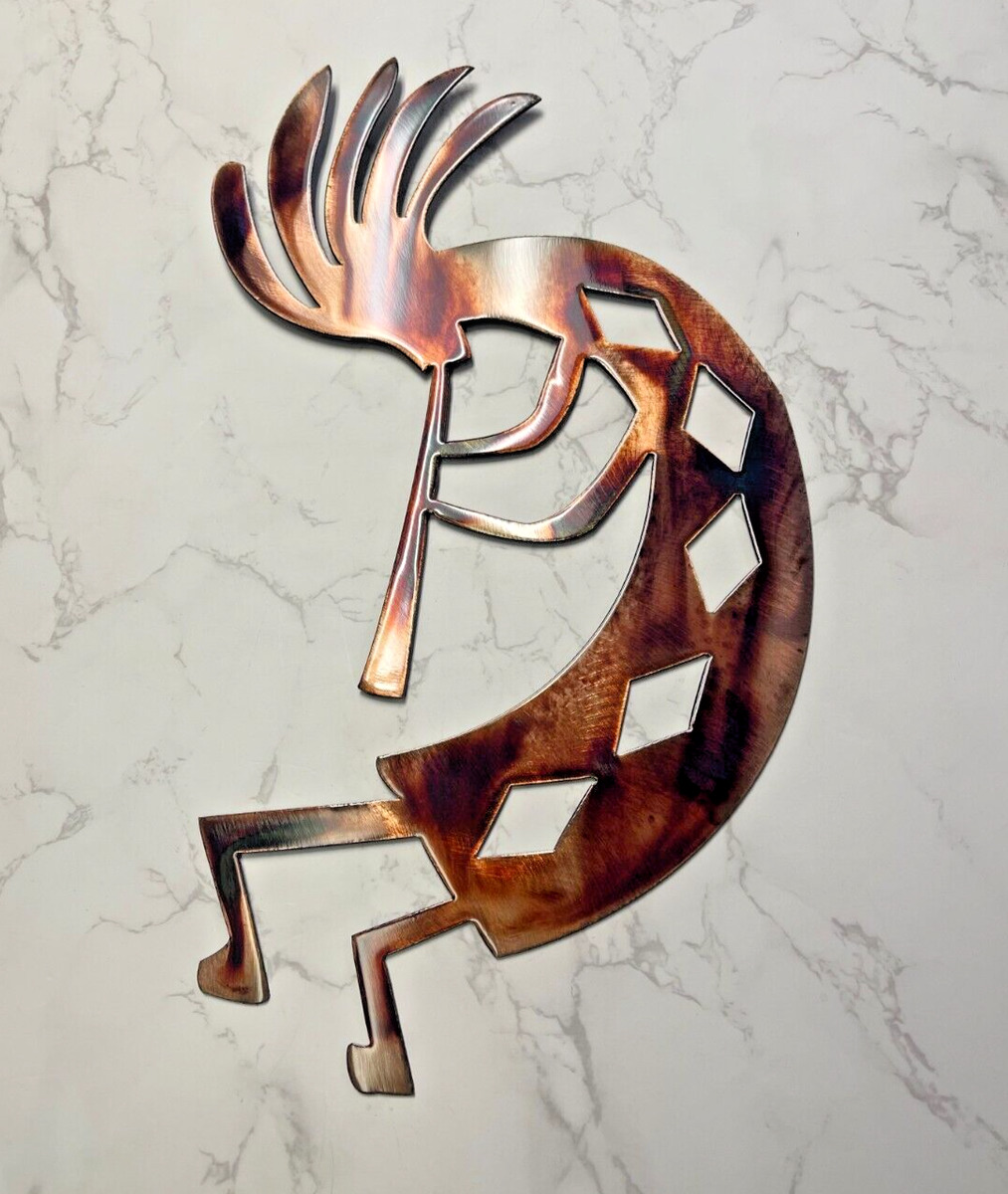The image depicts a bronze-colored, flat metal sculpture with dark tortoise shell staining, representing a Kokopelli figure, a deity from Native American culture known for playing a flute. The figure is mounted on a background resembling white marble with intricate gray veins, giving a realistic photographic representation. The Kokopelli is shown in profile with its body curved into a reverse C, legs angled downward, and feet at the bottom. Its head bends forward, featuring five large strands resembling feathers or hair flowing backwards, creating a dynamic sense of movement. The figure’s torso displays a pattern of five cut-out diamond shapes. Both arms are extended toward the front, holding a long, narrow flute that widens at the bottom near its mouth, adding to the impression of a musician deeply immersed in their performance.